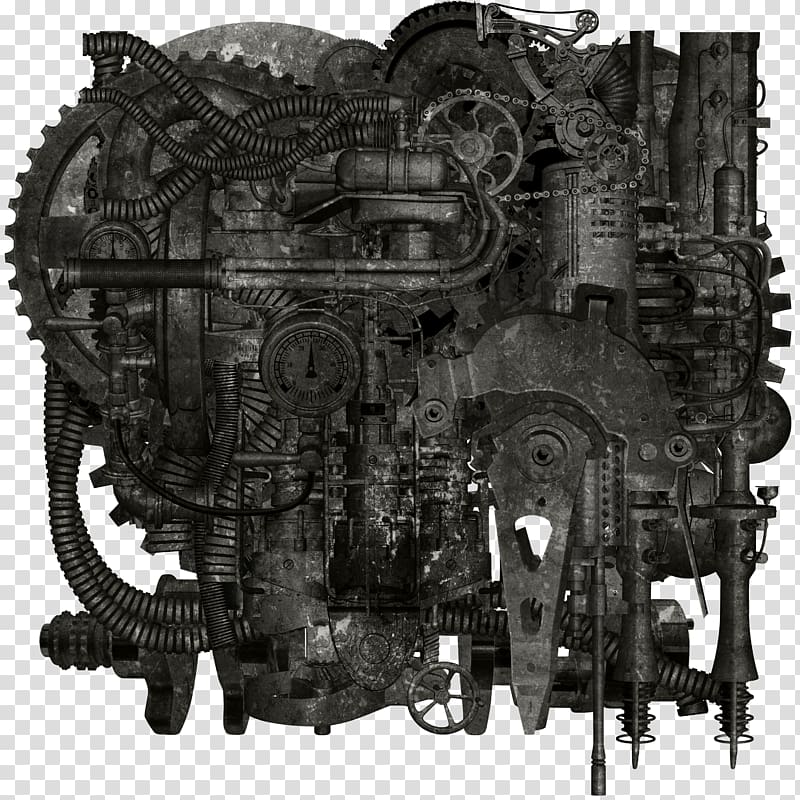In this detailed and complex image, we see a square-shaped contraption meticulously assembled from a myriad of metal components, including gears, levers, chains, springs, tubes, coils, cylinders, and pressure meters. The intricate configuration features exhaust parts, bolts, and various mechanical elements, all seemingly welded together. The metal parts predominantly display hues of blackish-gray with smudges of white and black, contributing to a steampunk aesthetic.

The background consists of a checkerboard pattern of blue and white squares, which frames the central mechanical structure. Hoses connect various parts of the contraption, mainly positioned towards the top left, middle, and bottom left sections of the image. The photograph is taken either from a top-down perspective or a side profile, presenting the elaborate mechanical assembly against the contrasting checkerboard backdrop. The overall impression is one of immense complexity, with a wealth of detailed components interwoven into a cohesive, visually striking piece.